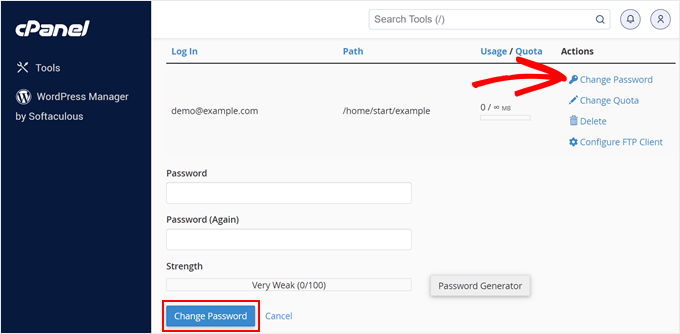The image depicts a user interface of an online application called cPanel. Prominently featured are two tools – a wrench and a screwdriver – accompanied by the word "Tools." Below this is the WordPress logo with the label "WordPress Manager by Softaculous."

The right area of the interface has a white background with black and blue text. At the top, there is a search tools bar, a bell icon, and a human icon positioned to the right. Directly beneath, in blue text, are column headers: "Login," "Path," "Usage Quota," and "Actions."

The main section showcases a user account with details:
- Login: demo@example.com
- Path: /home/start/example
- Usage Quota: 0/∞ MB

Under "Actions," there is a top entry marked by a red hand-drawn arrow highlighting options: "Change Password," "Change Quota," "Delete," "Configure FTP Client."

On the lower left, adjacent to a blue panel, there are two password fields labeled "Password" and "Password (Again)," both featuring entry boxes. The password's strength is indicated as "Very Weak (0/100)." To the right, there's a "Password Generator" button. Below this, a blue "Change Password" button is outlined in red, with a "Cancel" button to its right.